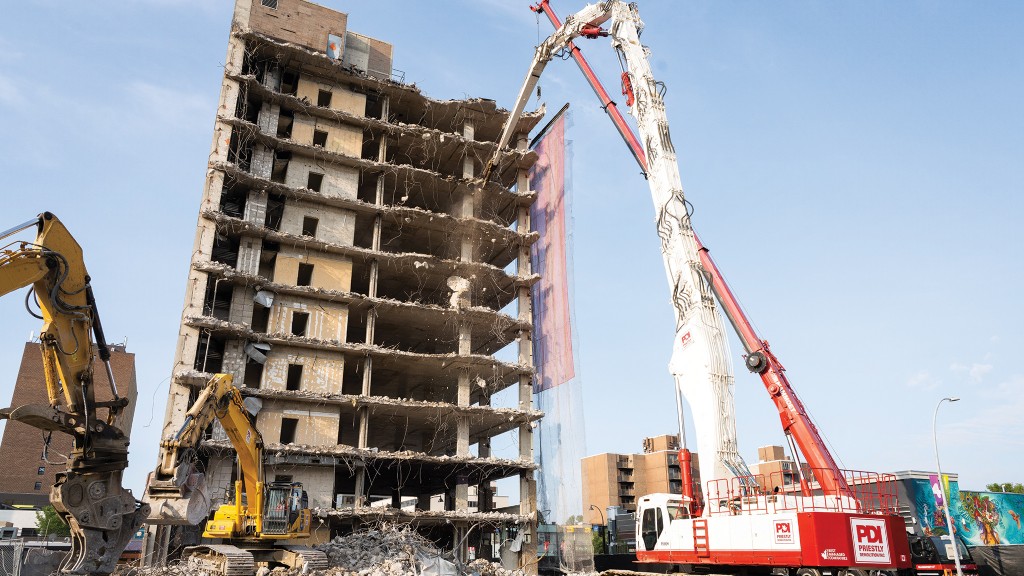The photograph captures a realistic, horizontally oriented scene of a building in the process of demolition on a bright, sunny day with a clear blue sky and few clouds. The building, approximately 10 to 12 stories tall, is already gutted and has been partially torn down, revealing the skeletal framework of concrete blocks, exposed stairwells, support beams, and floors stripped of windows and doors. Centered prominently in the foreground is a white and red, long-armed excavator, branded with "PDI Priestley," actively dismantling the building, its arm almost as tall as the structure itself. Surrounding the main excavator are additional pieces of heavy machinery, including two yellow excavators on the left. Rubble from the demolition is scattered at the base of the structure, and in the background, other city buildings stand, highlighting the urban setting. The image is of high quality and captures the vibrancy and details of the demolition in progress.